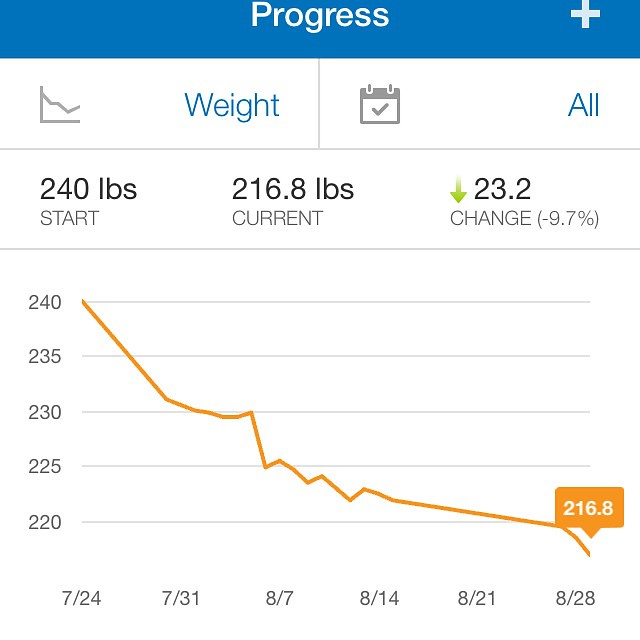The image is a detailed color screenshot taken from a weight loss app, displayed in a square format. Across the top, there is a horizontal dark blue bar with the word "Progress" in white text and a plus symbol on the top right side. Below this bar, two items are noted: "Weight" on the left side and "All" on the right, both in blue text with small graphic icons beside them.

Underneath these items lies a line of statistics: on the left, "Start" reads 240 pounds; in the center, "Current" reads 216.8 pounds; and on the right, "Change" is noted as -9.7% (down 23.2 pounds) with a down arrow symbol. The primary focus of the image is a bar graph situated towards the bottom portion, illustrating weight changes over time. Dates are marked along the bottom axis spanning from "7/24" to "8/28".

The graph itself tracks the user's weight from an initial 240 pounds, with a downward-sloping orange line indicating the weight loss progression, culminating at 216.8 pounds, which is highlighted in orange at the bottom right. The chart is grid-based with dates on the horizontal axis and weights on the vertical axis, set against a backdrop featuring colors like white, orange, black, blue, and gray. The app's interface appears well-structured, merging various design elements to effectively track and display the user's weight loss journey.